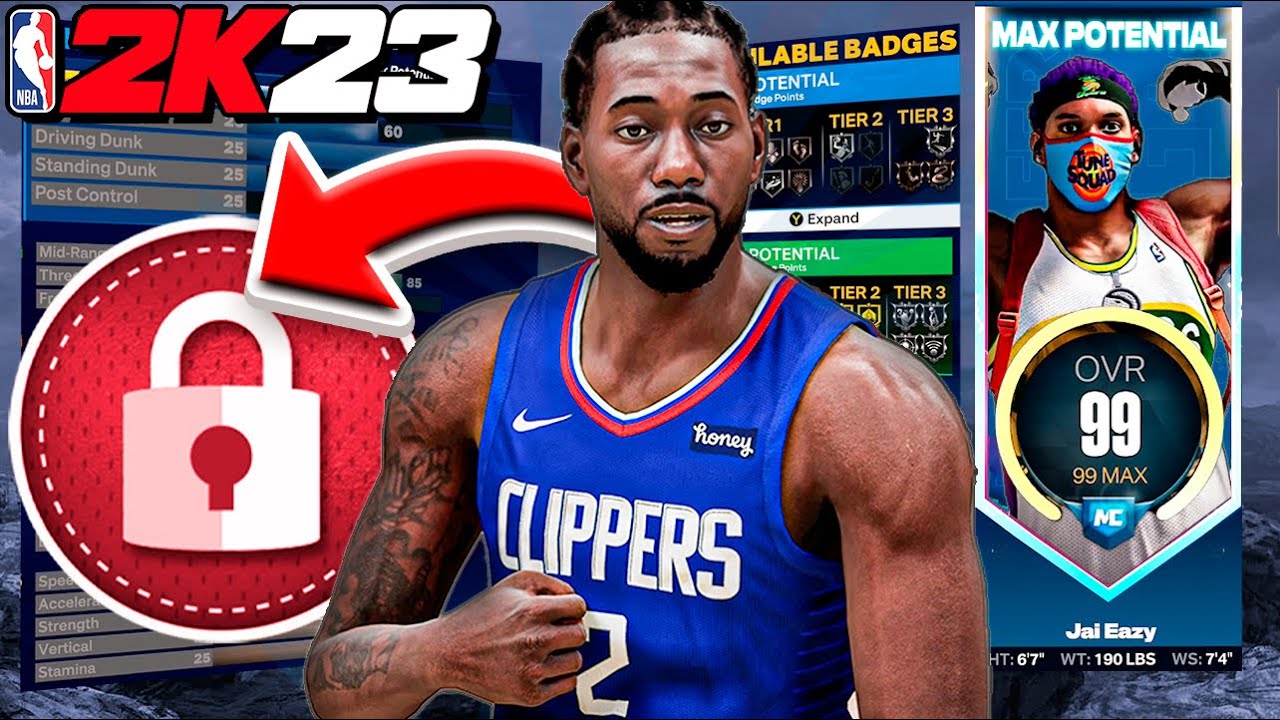A screenshot from the NBA 2K23 game illustrates a dynamic scene against a stormy gray background. In the upper left corner, the iconic NBA emblem is prominently displayed, split vertically into blue and red halves, with a white silhouette of a player holding a basketball. Below the emblem, "NBA" is written in white text, followed by "2K23" in bold, where "2K" is particularly emphasized before more subdued "23".

Dominating the center of the image is an African-American male basketball player dressed in a vivid blue Clippers jersey. The jersey is accented with red and white trim around the neck, featuring a Nike logo on the right shoulder and a white "Honey" sponsor logo on the left. Prominently across the chest, "Clippers" is written in white text, with the number "2" below it. The player, with short black hair, a neatly groomed black beard, and a mustache, gazes forward with his mouth slightly open. His right arm is lifted to his chest, revealing detailed tattoos extending from his shoulder to his forearm. Behind him, digital elements such as scoreboards, tiers, badges, and potentials are faintly visible, adding depth to the scene.

To the right, a slimmer rectangular strip features another African-American player dressed in a distinct white jersey with green and yellow trim and a face mask emblazoned with "Tune Squad". This player's arms are raised high, flaunting his biceps. Written across the top in white text is "Max Potential", and in a circular badge in front of his chest, detailed stats are displayed, reading: "OVER 99", "99", "Max MC", "J Easy", "Height 6'7", "Weight 190 Pounds", "WS 7'4".